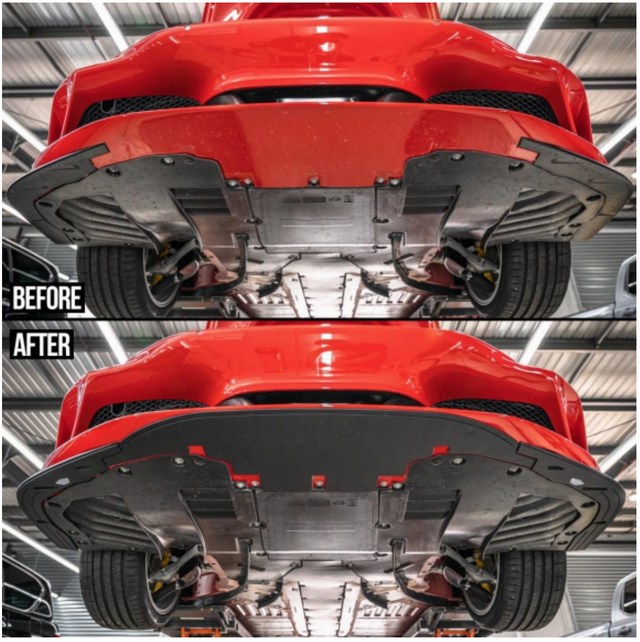The image is a detailed, indoor, photographic comparison showing the underside of a red sports car before and after a modification. The top photo, labeled "before" on the lower left corner, features an intricate, cherry red underside complete with visible mechanical parts, such as ribs and suspension, framed against a warehouse ceiling backdrop. Two wheels are visible towards the back. The bottom photo, labeled "after" in the upper left corner, showcases the same-view but with the entire underside now sleekly painted black. The only significant change between the two photos is the color transformation from red to black, giving the car a more polished appearance. Both images are set against a background of industrial elements and consistently show the gray metallic components of the car's frame.